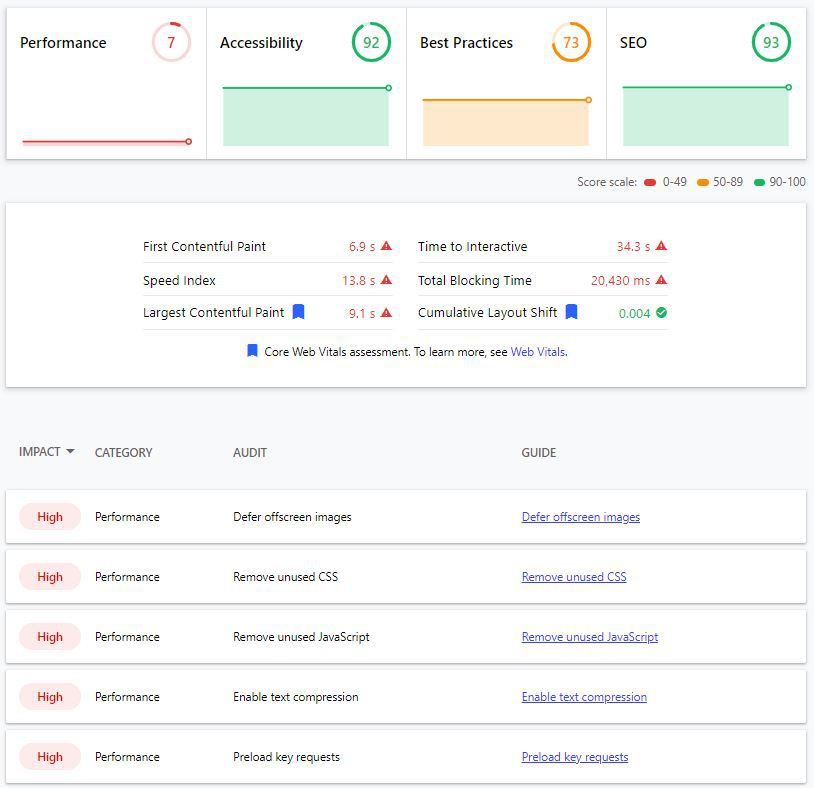The image depicts a web audit interface evaluating different aspects of a website's performance. There are four horizontally aligned white boxes, each assessing a distinct category:

1. **Performance**: This box shows a score of **7** encapsulated in a red circle, which has a darker red hue along its edges while the rest of the circle is a lighter red. Below the score, there is a red progress bar.

2. **Accessibility**: This metric scores **92** and is enclosed in a green circle predominated by a dark green shade, with a segment in light green. A horizontal progress bar underneath mirrors these green tones, starting darker and transitioning to light green.

3. **Best Practices**: The score here is **73**, displayed within a gold circle. Beneath it lies a progress bar in gold, featuring variations of lighter gold along its length.

4. **SEO**: This category boasts a score of **93**, highlighted within a nearly fully dark green circle, paired with a dark green band below it, transitioning into light green in the rest of the bar.

Below these boxes is a detailed performance section, featuring two critical metrics:
- **First Contentful Paint**: Listed as **6.9 seconds**, marked with a yellow triangle containing an exclamation point.
- **Speed Index**: Recorded at **13.8 seconds**, also flagged with a yellow triangle and an exclamation point.

This interface provides a comprehensive overview of the website's current operational status across multiple performance fronts.